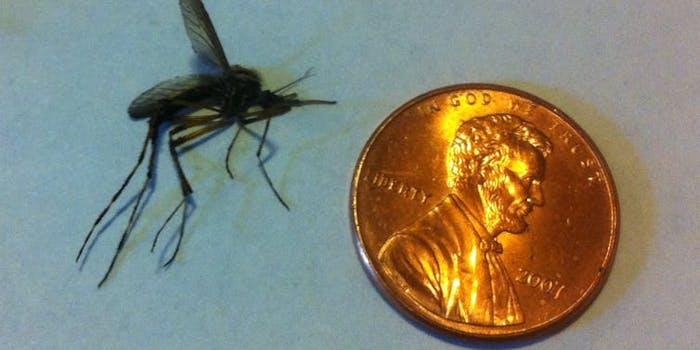The image features a highly detailed close-up of a bright, shiny copper penny resting on what appears to be a grayish-blue, flat surface, possibly a table or countertop. The penny, positioned in the bottom right corner, prominently displays the inscriptions "In God We Trust," "Liberty," and the year "2007," along with President Lincoln's profile. To the top left of the image, there is a black, dead insect that appears to be a mosquito, with two see-through wings, two antennae, and five legs. The comparison visually highlights the size difference between the penny and the mosquito, with no additional text or objects visible in the image. The setting seems to be indoors, suggested by the lighting and nature of the background.